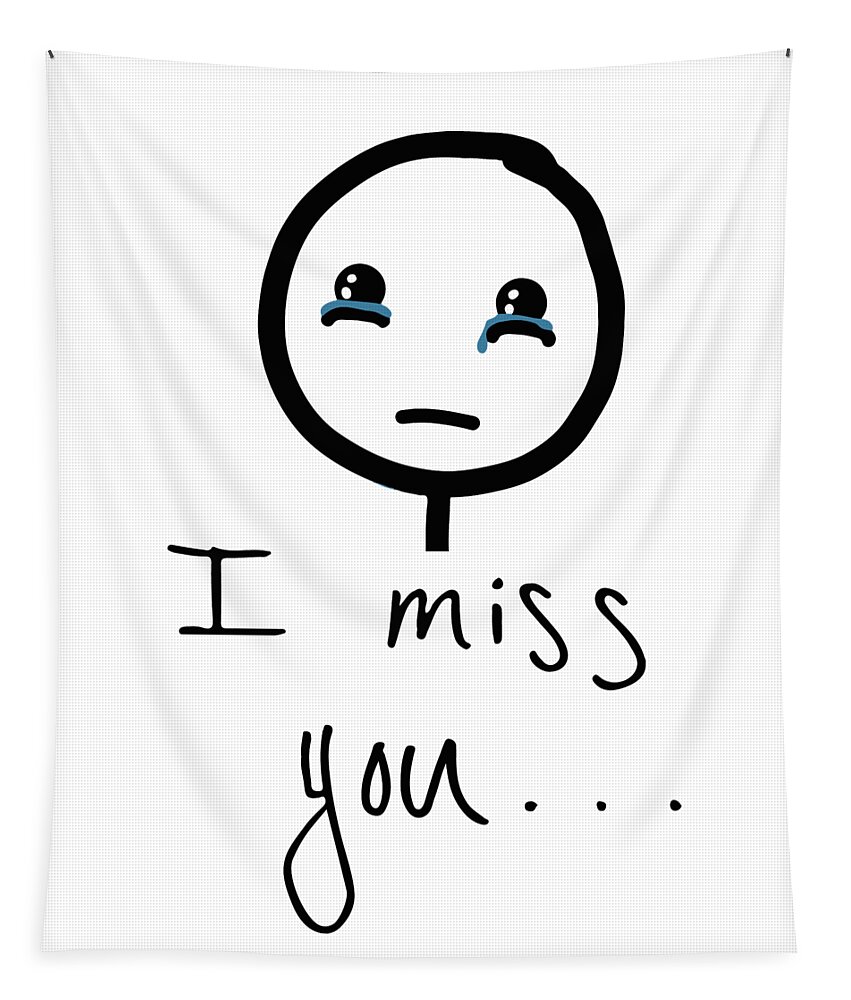The image depicts a white sheet or possibly a pillowcase with a subtle, almost plaid-like detailing. The center of the fabric features a simple yet poignant sketch of a stick figure's head, comprising a circle for the head, two large black eyes with tiny white highlights, and a tear falling from the left eye. The tear is illustrated by small blue and black lines extending horizontally from each eye. The stick figure has a slight frown, represented by a gently curved black line. Below this sorrowful face, the words "I miss you..." are written in black lettering. The cloth appears to be pinned in the top right and left corners.